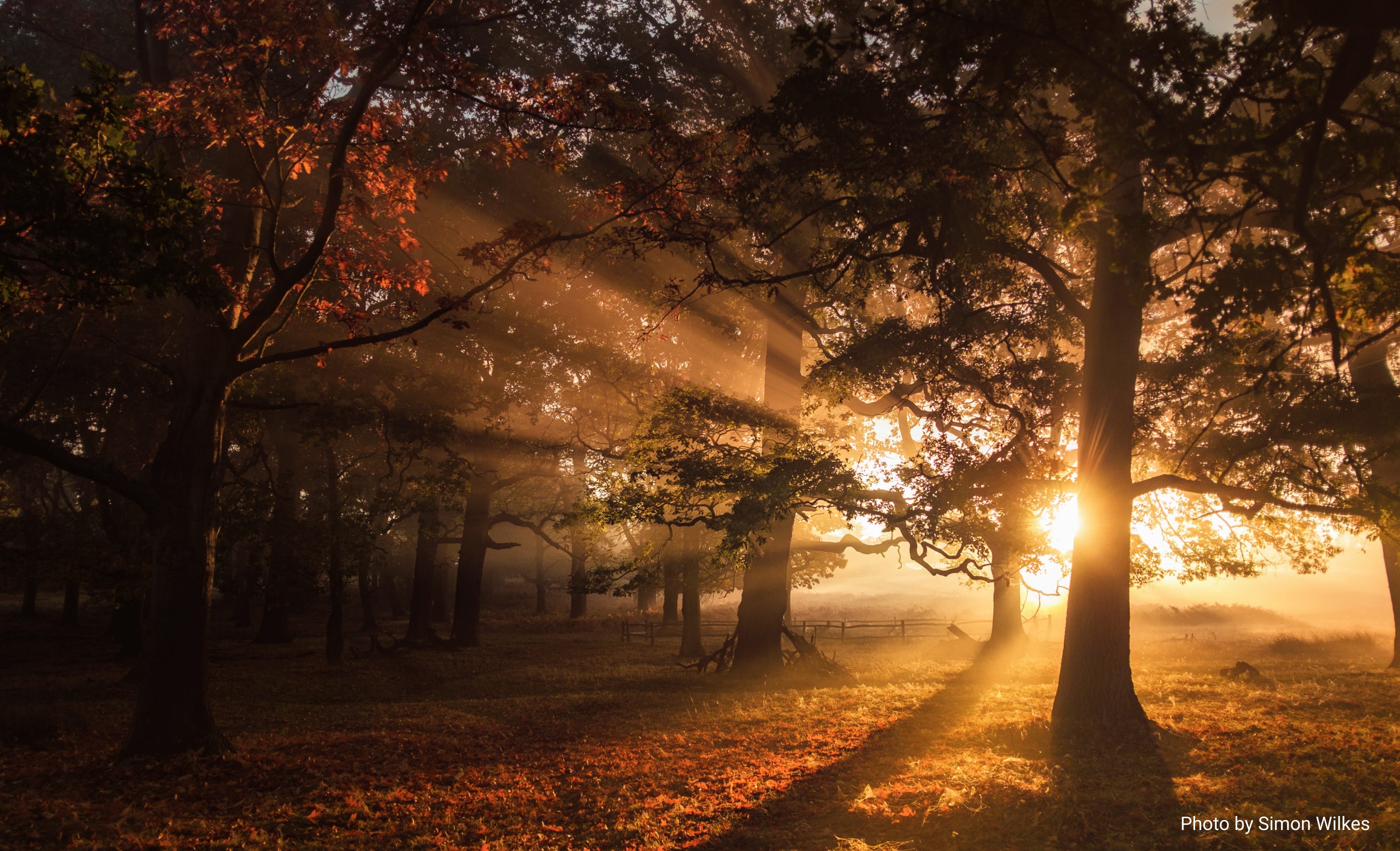This photograph captures a serene sunset scene through a sparsely wooded area, likely on private property. The mature trees, free of undergrowth, stretch their leafy branches widely, casting long shadows on the orange-hued ground. The low sun is positioned towards the right of the image, emitting warm yellow light that filters through the trees, creating a striking interplay of light and shadows. Sunbeams, refracted by dust in the air, extend from right to left across the scene. In the background, you can discern a faint split rail fence hinting at a large backyard or farm property, possibly bordering a less dense forest. The sky peeking through the trees appears gray, enhancing the dramatic contrast with the almost black trunks, some of which have a slight orange tinge on the left. A watermark in the bottom-right corner credits the photo to Simon Wilkes.